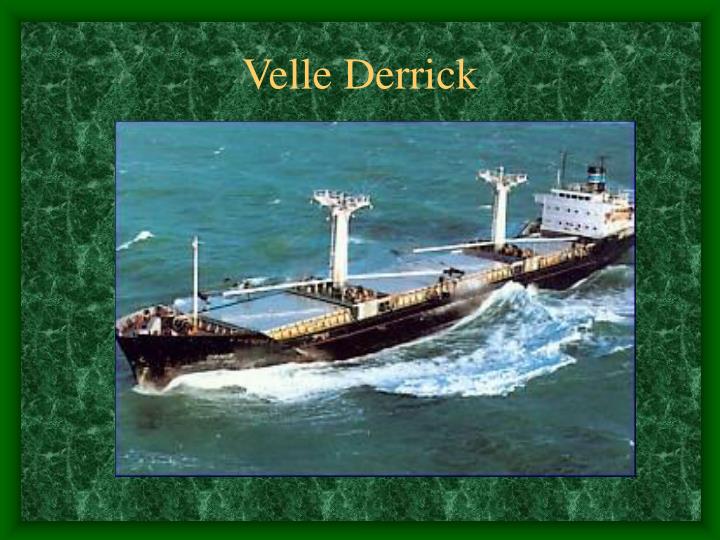The image features a large black ferry, prominently displayed in the center and moving through choppy waters, creating visible waves. The ferry, which could be transporting people or goods, has distinctive white trim, white cabins at the back, and two large white masts along with a smaller mast at the front. The vessel's intricate details include a black stack behind the cabin and a bustling deck where people might be observable. Surrounding this central image is a forest green square background, textured and bordered by a darker green hue. Above the ship in this green section, yellow text spells out "VELLE DERRICK," which is likely the name of the ferry.